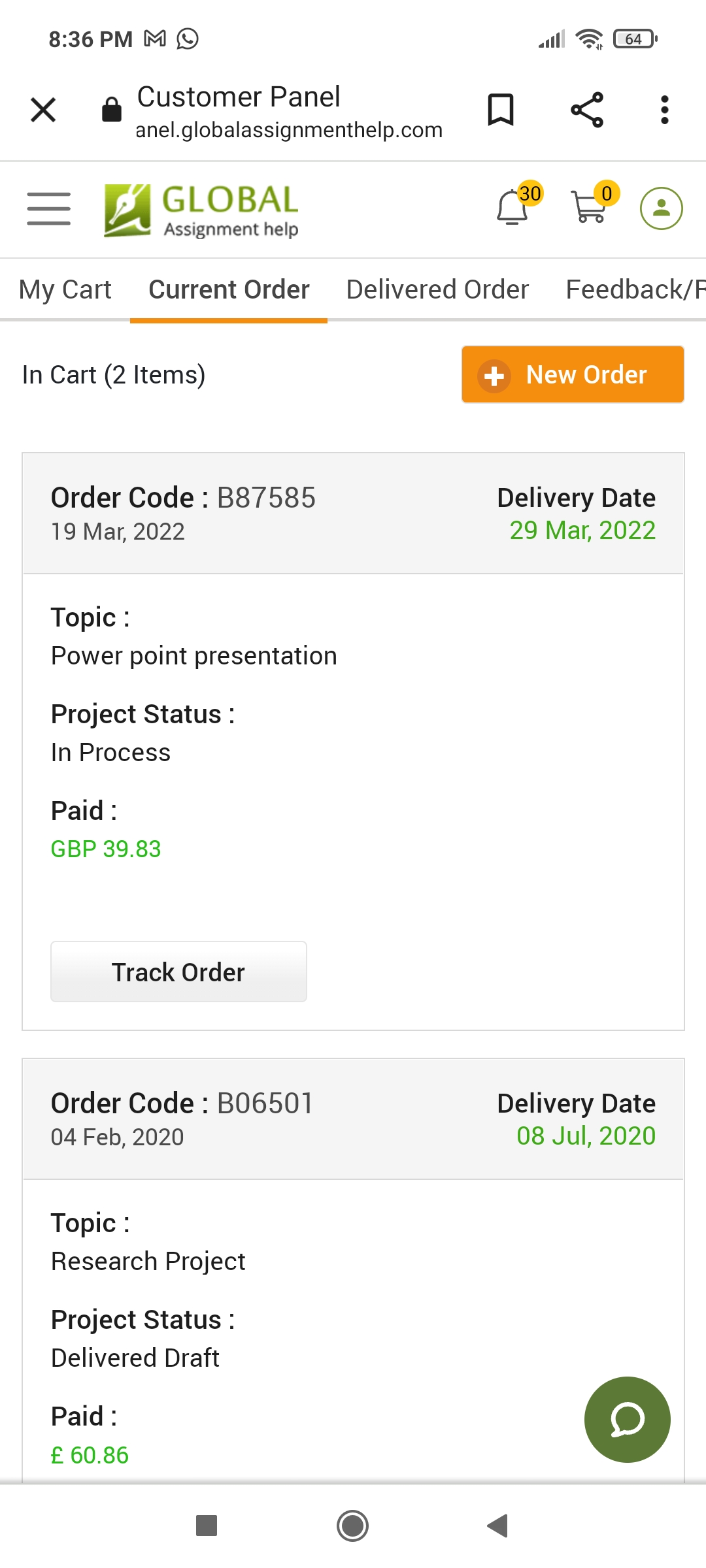A smartphone screenshot displaying a detailed interface of a customer panel on a white background. At the top left, it shows the time "8:36 PM" next to the Google Mail logo (an outlined "M") and the WhatsApp logo (a speech bubble with a phone inside). On the top right, icons indicate almost full cell phone coverage, full Wi-Fi signal, and a 64% battery level.

The next line features three icons: a black "X," a black lock, followed by the text "Customer Panel." Adjacent to this are a website address bar, bookmark icon, "weird thing with lines" (likely a menu icon), and three vertical dots (more options).

Below this toolbar, the interface presents several navigation items: "Global" highlighted in green, "Assignment Help" in black, a bell icon with the number "30," a shopping cart icon with "0," and a profile icon.

Further down, it states "My Cart," "Current Order," "Delivered Order," and "Feedback/F." The section underlines that there are "In Cart: 2 items" followed by an orange button with white text and a plus sign reading "New Order." Below that, a gray background text indicates an order "Order Code: B87585" with a delivery date range. Specifically, the delivery dates are mentioned as March 19, 2022, and March 29, 2022.

The details section specifies the topic as "PowerPoint Presentation Project," status marked "In Status," payment labeled "Paid," amounting to "GDP 3983." The order is being tracked, with the research topic for a PowerPoint presentation.

(Note: The colors and icons mentioned might indicate an educational or assignment assistance app, highlighted by the text such as "assignment help" and "research topic.")